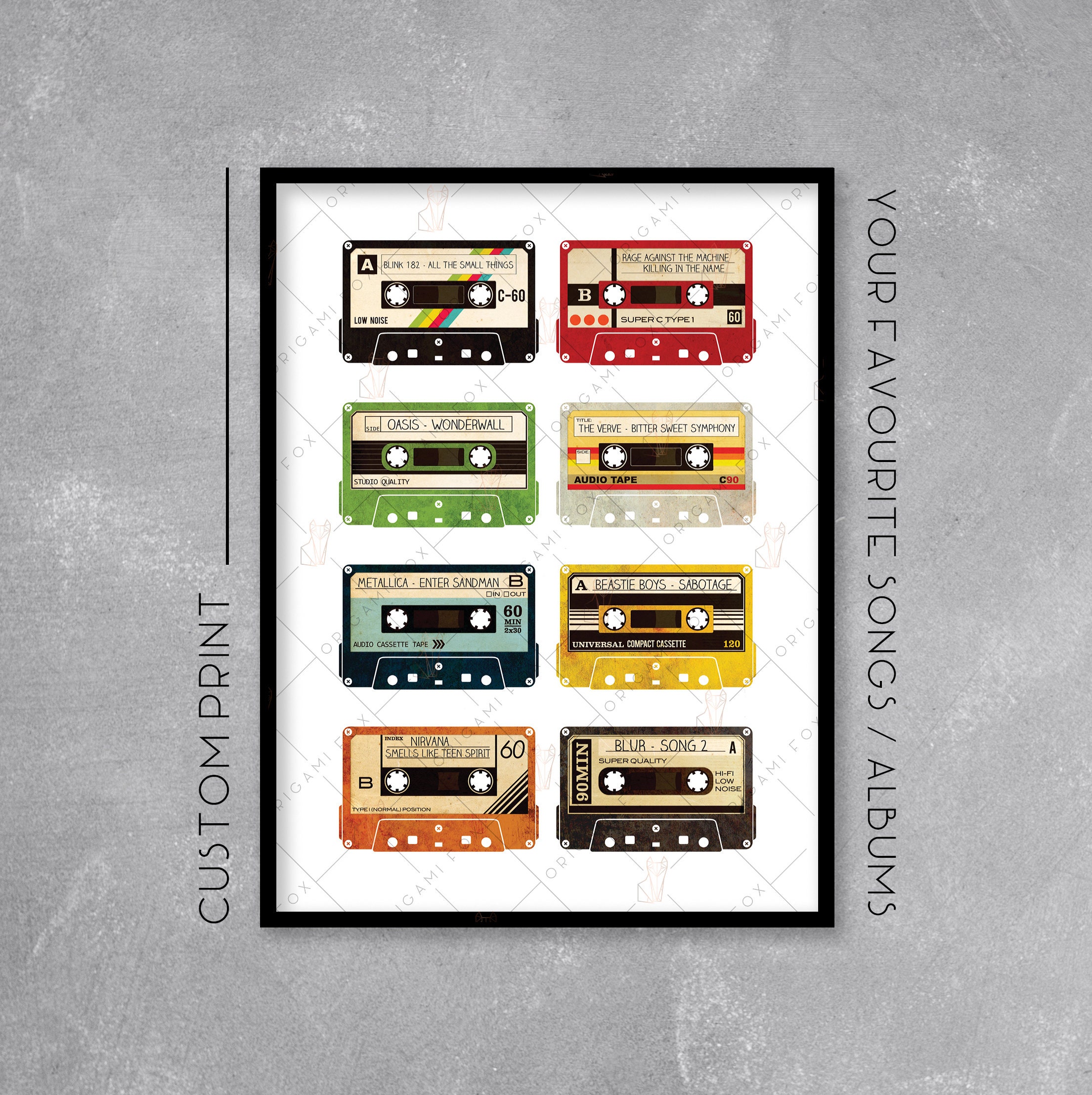The image portrays a print designed as wall art, featuring eight retro-style cassette tapes against a dark grey background. Vertical text flanks the sides, with "custom print" on the left and "your favorite songs/albums" on the right, suggesting personalized options for print. Each cassette, styled with different colors and labels like C60 and B60, showcases iconic songs and albums, emphasizing a vintage aesthetic. Notable titles include Blink-182's "All the Small Things," Oasis' "Wonderwall," Metallica's "Enter Sandman," Nirvana's "Smells Like Teen Spirit," Rage Against the Machine's "Killing in the Name," The Verve's "Bittersweet Symphony," Beastie Boys' "Sabotage," and Blur's "Song 2." A watermark, likely of the company offering the custom prints, is present, indicating this as an advertisement for personalized wall art.